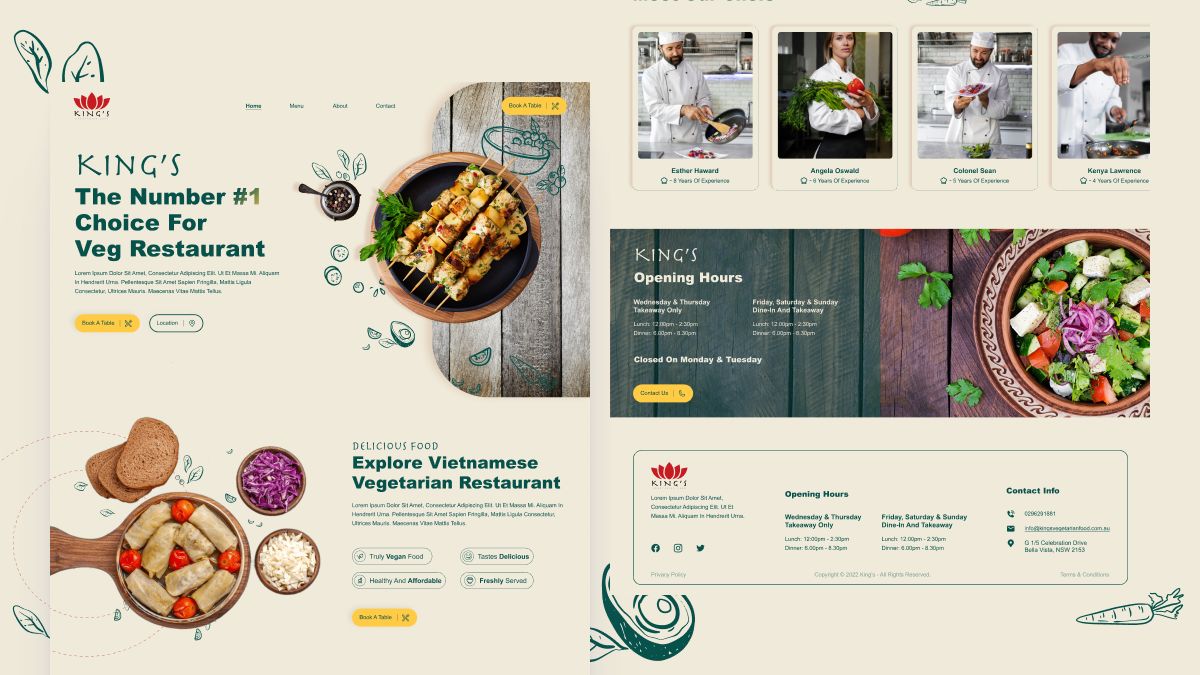**Caption:**
This digital poster showcases King's, the number one choice for a vegetarian restaurant specializing in Vietnamese cuisine. The webpage's title, displayed in blue, reads "King's: The Number One Choice for Veg Restaurant." The background color of the poster is beige, adorned with green text, numerous photographs, and a chart on the right side.

At the top right corner, there's a red lotus flower icon representing King's. Adjacent to the title is a vivid image of a bowl filled with four meat skewers garnished with a mint leaf. Directly below the title, another headline, "Explore Vietnamese Vegetarian Restaurant," captures attention. To the right of this text, a visual feast includes dumplings, Roma tomatoes in a wooden bowl, three slices of bread, and two bowls of condiments.

On the right side of the poster, the top row features photographs of four chefs: Esther Howard (8 years of experience), Angela Oswald (9 years), Colonel Sean (9 years), and Kenya Lawrence (4 years). Each chef’s name and experience are clearly mentioned.

Beneath the chefs' photos is a banner displaying King's opening hours and a contact button. Adjacent to this banner is a delectable image of a vegetable dish consisting of cucumbers, red onions, and chopped tomatoes.

Below this, a detailed chart outlines King's opening hours, lunch hours, dessert hours, dining and takeaway times, as well as their social media profiles (Facebook, Instagram, and Twitter). The contact information, including a phone number, email address, and physical address, is provided at the far right of the chart. The restaurant is located in New South Wales, Australia.